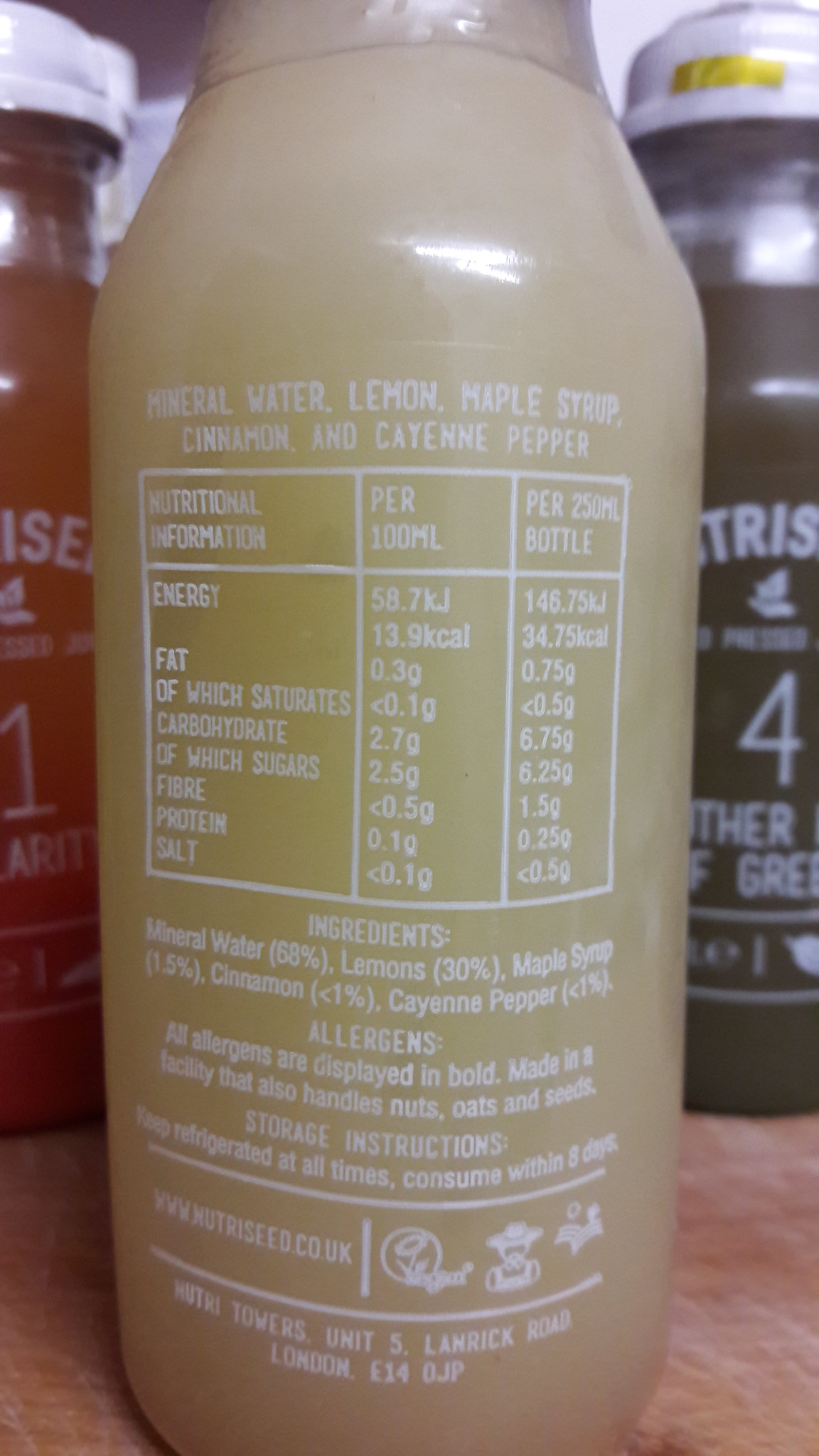The image features three bottles arranged against a backdrop. On the far left, a bottle is partially visible, and another bottle stands at the back right. Taking center stage is a clear bottle containing a white liquid. This bottle has a prominent label with white text that reads: "Mineral Water, Lemon, Maple Syrup, Cinnamon, and Cayenne Pepper." Below this text, the label is divided into three columns. The column on the left is titled "Nutritional Information." The label appears to provide detailed content about the beverage inside the bottle.